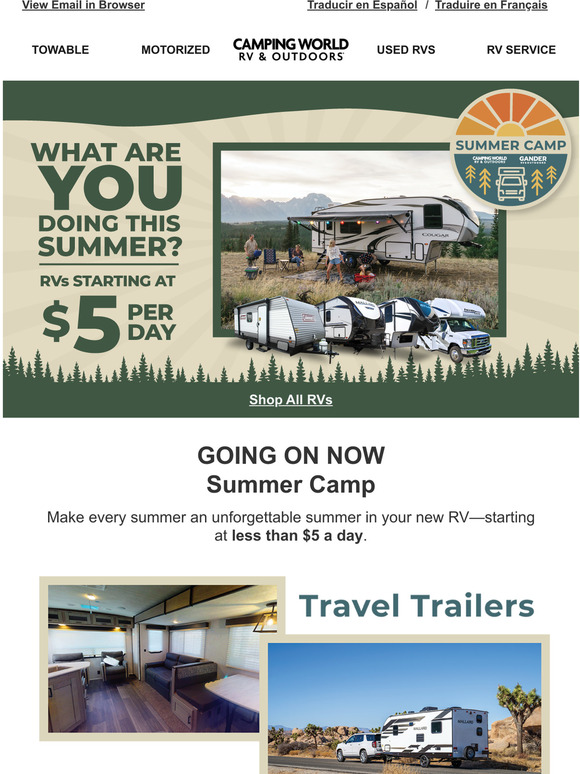Website Screenshot for Summer Camping Promotion: Detailed Description

The screenshot captures a colorful, engaging website dedicated to promoting summer camping activities, particularly focusing on RV adventures. At the top of the page, there are options to view content in Spanish ("Traducir en Español") and French ("Traduire en Français"), alongside quick links for email and browser settings.

The primary sections of the site advertise various RV categories, including "Towable," "Motorized," "Camping World," "RV and Outdoors," "Used RVs," and "RV Service." A prominent, inviting headline asks, "What are you doing this summer?" followed by a persuasive offer: "RVs starting at five dollars per day."

One of the key visual elements is a vibrant image showing a family enjoying an outdoor cookout next to their parked RV. Behind them, there are four more RVs neatly arranged, emphasizing the communal and expansive nature of RV camping.

Below this image, there is a call-to-action button, "Shop All RVs," drawing visitors further into the website. The background features a soothing brown color, with green accents at the top and bottom, supplemented by tree illustrations that evoke a natural, camping environment.

Further down, there's a banner highlighting the current promotion: "Make every summer an unforgettable summer in a new RV starting at less than five dollars a day." This section promotes travel trailers, showcasing images of a trailer being towed and the detailed, cozy interior of another trailer. The inside view reveals a homely setting with window shades drawn, wood fixtures, comfortable seating including a couch and chairs, and a dining table, all ready for a summer adventure.

This detailed, visually captivating website layout not only promotes summer camping but also invites viewers to explore the joys of RV travel, enticing them with affordable and memorable summer experiences.